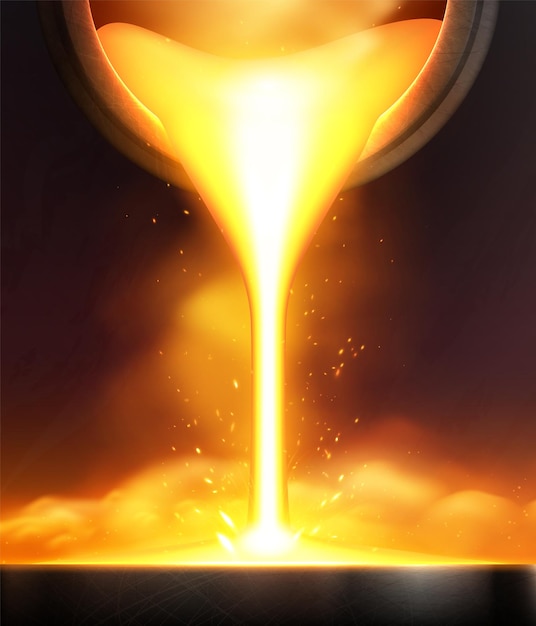In this digitally rendered artwork, a surreal scene unfolds where a large cream-colored cup hovers against a nearly darkened sky, pouring a stream that intriguingly mimics both creamy coffee and molten lava. The fluid, radiating with bright yellows, oranges, and whites, cascades down from the cup's lip, creating a dynamic splash that resembles a wave upon impact. Beneath this wave, a distinctive black or gray border gives the impression of a solid land surface, contrasting with the luminous flow above. The sky serves as a striking backdrop, adding depth and emphasizing the extraordinary blend of elements in this imaginative composition.